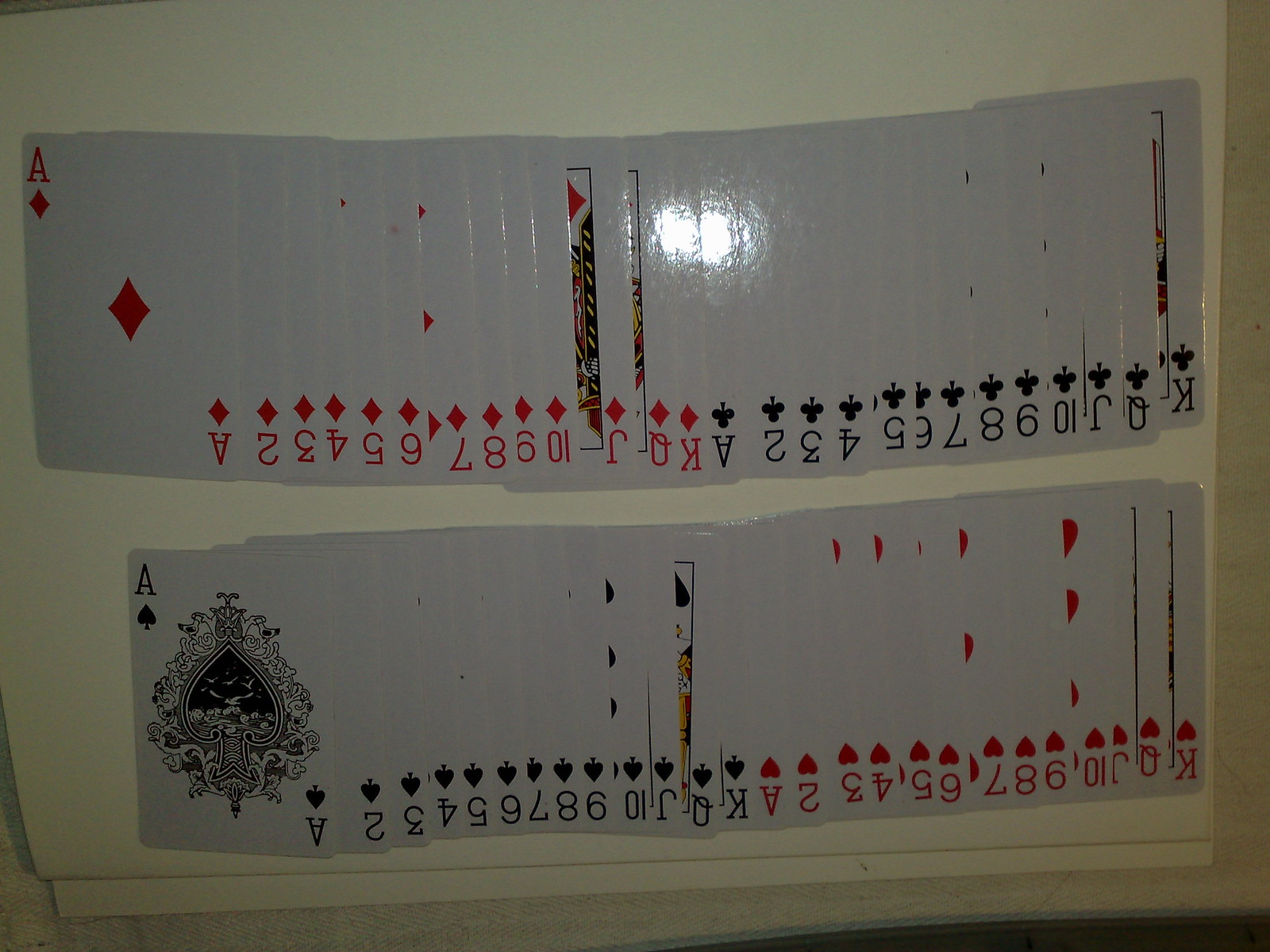The image depicts a neatly arranged deck of playing cards, each card slightly spread out to reveal its face value and suit. The entire deck is meticulously mounted on a piece of cardboard, with a laminated or film covering securing the cards in place to prevent any movement. This arrangement allows viewers to easily identify each card, from the Ace of Spades to the King of Diamonds and the Queen of Hearts. The setup might be part of a school project, an educational tool for learning card games, or a creative decoration. The image appears to be upside down, suggesting it was photographed from an angle that shows the cards lying flat on a table or countertop. The careful presentation and lamination hint at an effort to preserve and display the cards in an organized and visually appealing manner.